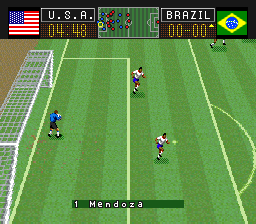This small screenshot captures a nostalgic moment from an old vintage soccer video game. Dominating the scene is a digitally rendered green soccer field, complete with the characteristic white lines that demarcate the playing area, including the goal boxes and the center circle. On the left side of the screen stands a white goal with a net, vigilantly guarded by a goalie in a blue jersey. The stance of the goalie indicates readiness, situated right in front of the net.

The image showcases a match between two national teams: Team USA and Team Brazil, as identified by the flags displayed on their respective sides. A digital scoreboard at the top of the screen reveals that there are 4 minutes and 48 seconds remaining in the game, and the current score stands at 0-0, suggesting a tightly contested match. Positioned in the center-top of the display is a mini-map that provides an overhead view of the field, showing the positions of all the players, aiding players in strategic gameplay. This screenshot encapsulates the classic charm of early video game graphics, bringing a wave of nostalgia for vintage gaming enthusiasts.